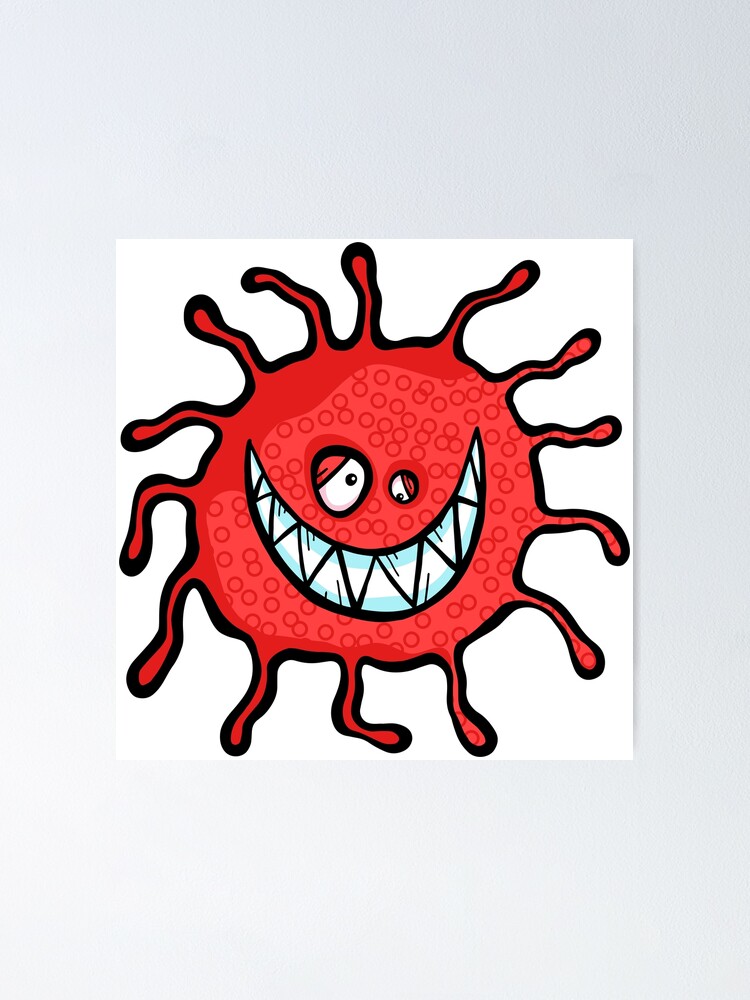The image is a vertically rectangular, two-toned artistic piece with a gray border that fades to nothingness on the left side, revealing a central white square. Within the white square, there is a vivid illustration of a red, monster-like figure that resembles a cartoon version of the COVID-19 virus. The creature is round with numerous red, squiggly, trumpet-like tentacles extending from its body, each unique in shape and length. The monster's face is quite expressive, featuring two eyes—one larger, looking straight ahead, and the smaller one glancing down. The eyes have red eyelids, white sclera, and black pupils. It has a wide, jagged grin filled with sharp, triangular teeth that interlock perfectly when closed. Small red circles are scattered throughout its body, adding to its intricate detail. The background behind the white square is a light blue hue, further emphasizing the central figure.